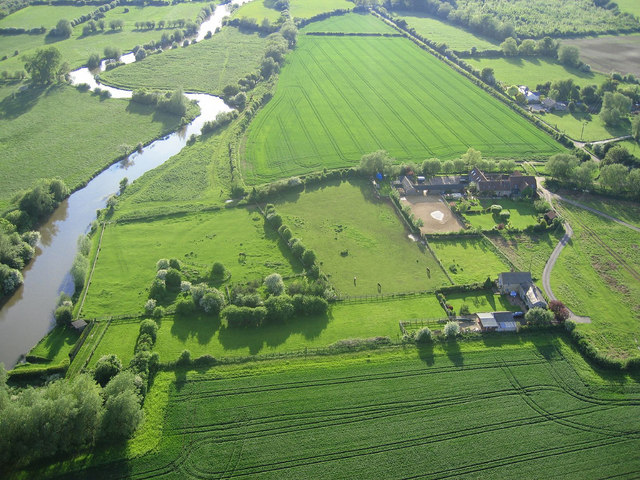An aerial shot, likely taken from a drone or small aircraft, showcases a vast, lush landscape of rural farmland. Dominated by neatly mown, green fields, the image highlights the various plot outlines, each bordered by trees, giving a sense of individual ownership within the expansive terrain. A serene stream meanders through the land, its surface reflecting the bright, sunny sky. Scattered throughout the area are a few sizable homes and farm buildings, some of which appear multi-story, indicating they might be the primary residences or main structures of the properties. The roads weave through this picturesque, well-maintained setting, which exudes a sense of tranquility and meticulous care. The abundance of grass, the vibrant greenery of the trees, and the clear organization of the farms under a brilliant sun collectively create a vivid and serene rural landscape.